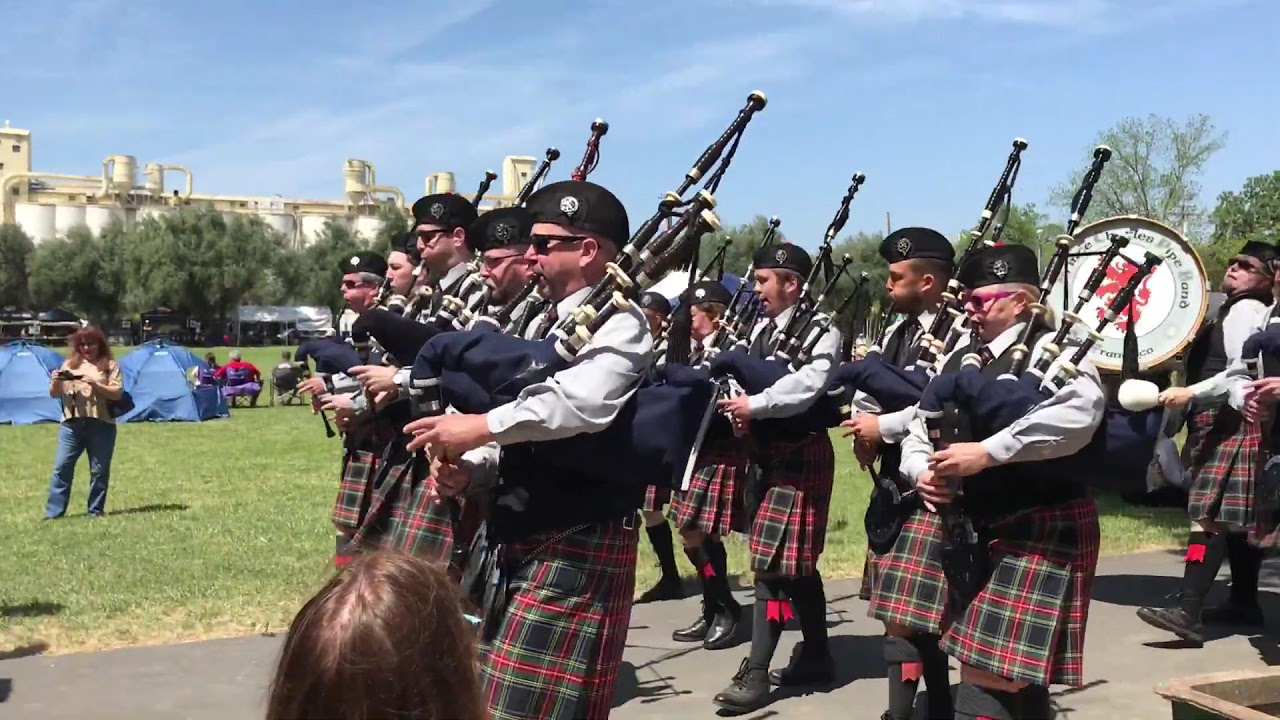In this vibrant color photograph, a parade is captured in landscape orientation, showcasing a traditional marching band as its central focus. The band members, all clad in classic Highland regalia, feature prominently with their blue, black, and white bagpipes. They don black berets adorned with a silver insignia, black vests over cream-colored long-sleeve shirts, black ties, and red, green, and black plaid kilts. Accentuating their attire, they wear black socks with red ribbons and matching black shoes.

The marchers proceed from the right to the left side of the image, immersed in their performance. Positioned on the right side of the frame, a drummer plays a large drum with two white, cloth-covered drumsticks; the drum itself is emblazoned with a red lion emblem encircled by the words "pipe band." In the foreground, a spectator's head offers a subtle framing to the scene, indicating the engaging atmosphere of the event.

In the background, a grassy park stretches out under a clear blue sky, dotted with blue tents and dotted with a few onlookers. Trees border the back of the park, with a large building faintly visible, contributing to a sense of place. The overall style of the photograph adheres to representational realism, capturing the detail, tradition, and camaraderie of the parade.